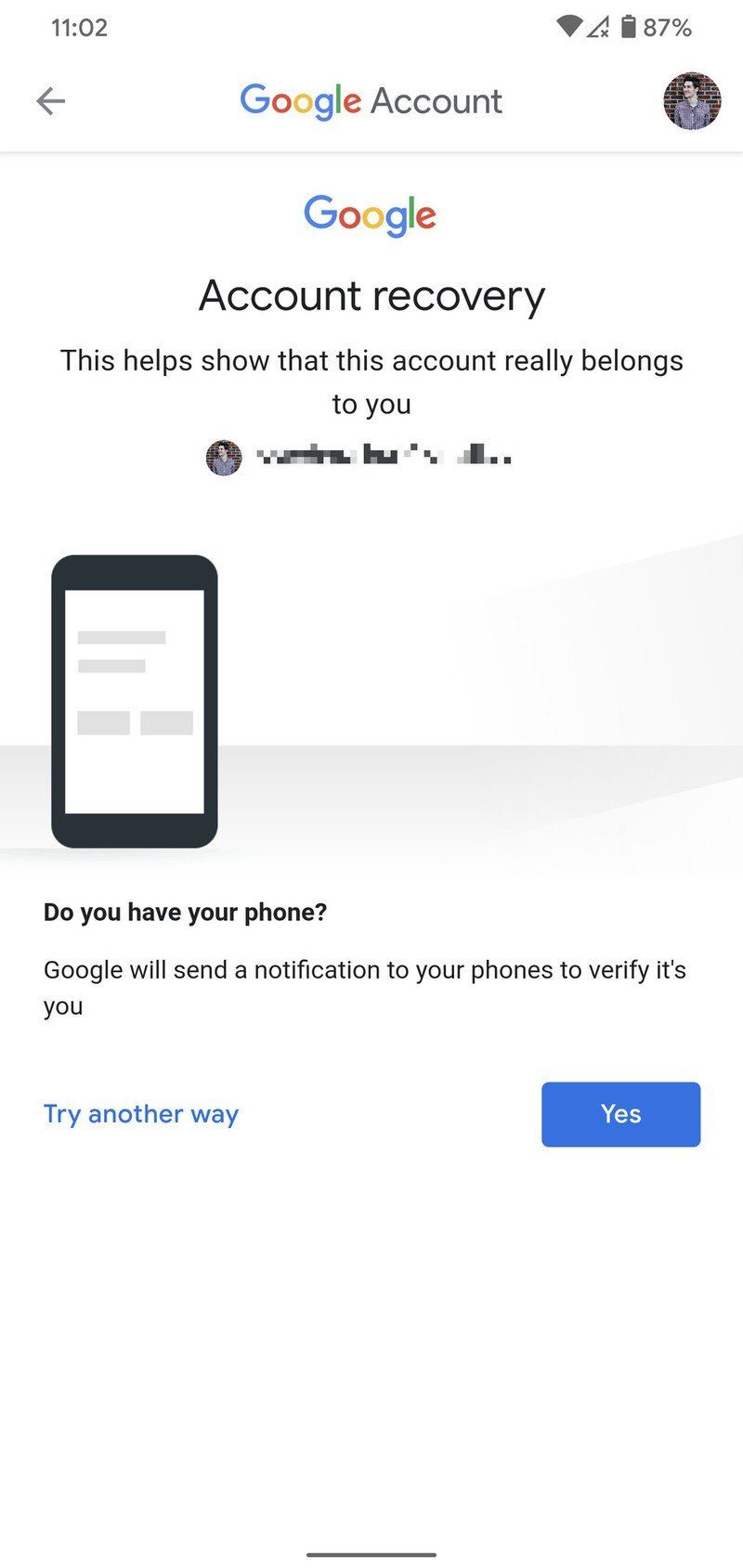This image depicts the Google Account recovery screen as viewed from a mobile device. At the top of the screen, the time is displayed as 11:02 AM on the left, while on the right, icons for Wi-Fi signal strength, cellular signal, and battery level at 87% are visible. 

On the bottom left corner, there is a gray back arrow for navigation. Central to the image is the Google logo accompanied by the word "Account." To the right of this, the user's profile picture can be seen. Below this header, the Google logo reappears with the title "Account Recovery," followed by an explanatory statement: "This helps to show that this account really belongs to you." 

The user's profile picture is shown again underneath this message, with the email address blurred to maintain privacy. Further down, an illustration of a mobile device is depicted alongside the question, "Do you have your phone?" Google explains that a notification will be sent to the user's phones to verify their identity. Below this, options are available to either press the "Yes" button to confirm possession of the phone or to try another recovery method.